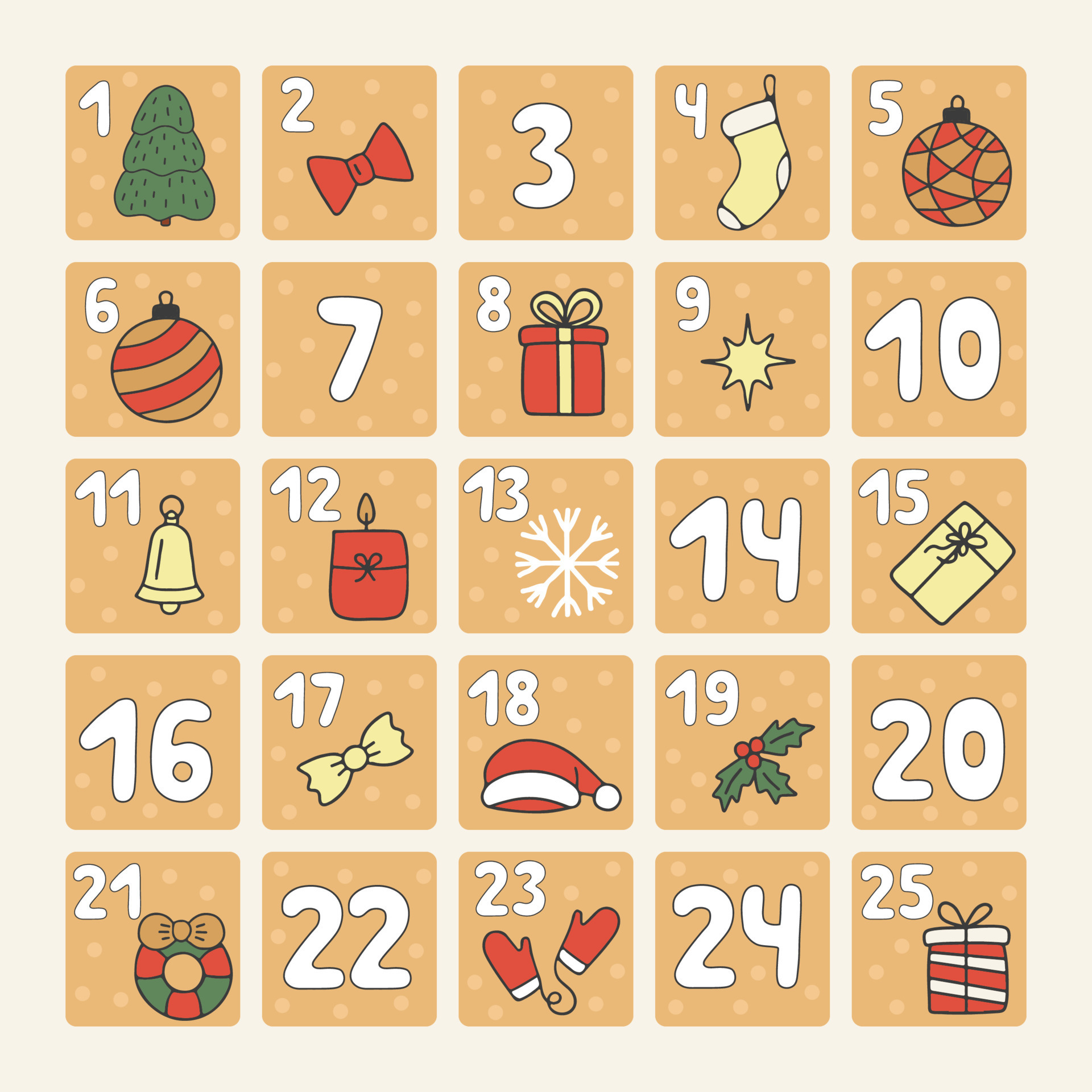The image depicts a Christmas-themed countdown calendar with numbered squares from 1 to 25, each adorned with various holiday symbols. The calendar is organized into five rows, with each row containing five squares. The squares themselves feature a festive color palette predominantly including orangey-browns, reds, greens, and yellows, with all numbers written in white. 

Day 1 showcases a Christmas tree, while Day 2 features a red bow. Day 3 is simply marked with the number 3. Day 4 highlights a stocking, and Day 5 displays an ornament with red and brown geometric patterns. Another striped ornament is shown on Day 6. Both Days 7 and 10 only have their respective numbers without any decorations. On Day 8, there is a gift box; Day 9 exhibits a star. Day 11 pictures a bell, followed by a red candle with a bow on Day 12. Day 13 shows a snowflake. A second present, white with a bow resembling a butterfly, decorates Day 15. The trend continues with another plain square for Day 14. Day 16 is empty, but Day 17 features another bow, similar in shape to bowtie pasta. The Santa hat rounds out Day 18, and mistletoe appears on Day 19. Days 20, 22, and 24 are again just numbered. Day 21 includes a wreath decorated with a brown bow. Red and white mittens connected by a string adorn Day 23, and finally, a red and white striped present with a black bow signifies Day 25.